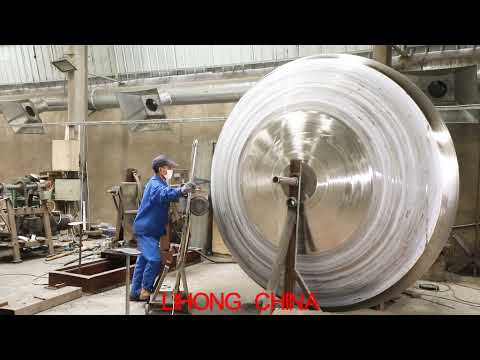This color photograph captures an industrial scene dominated by a concrete floor and wall, with an overlay of metal piping and vents running across the upper section. Positioned near the center left of the image, an Asian workman clad in blue work clothes—a jacket and pants—and a blue or gray baseball cap, is seen climbing a step stool. He is wearing a white medical mask and gloves, and his gaze is fixed on a large, shiny metallic disc positioned just to his right, which seems to be spinning on an axis with a steel bar running through its center. The man appears to be holding a tool or instrument up against the spinning disc, suggesting he's possibly polishing or cleaning it. The setting is cluttered with industrial machinery, metal pipes, lathes, and other metallurgical equipment. Black bands frame the top and bottom of the photograph, with bold red text at the bottom center reading "LHONG China, CHINA."